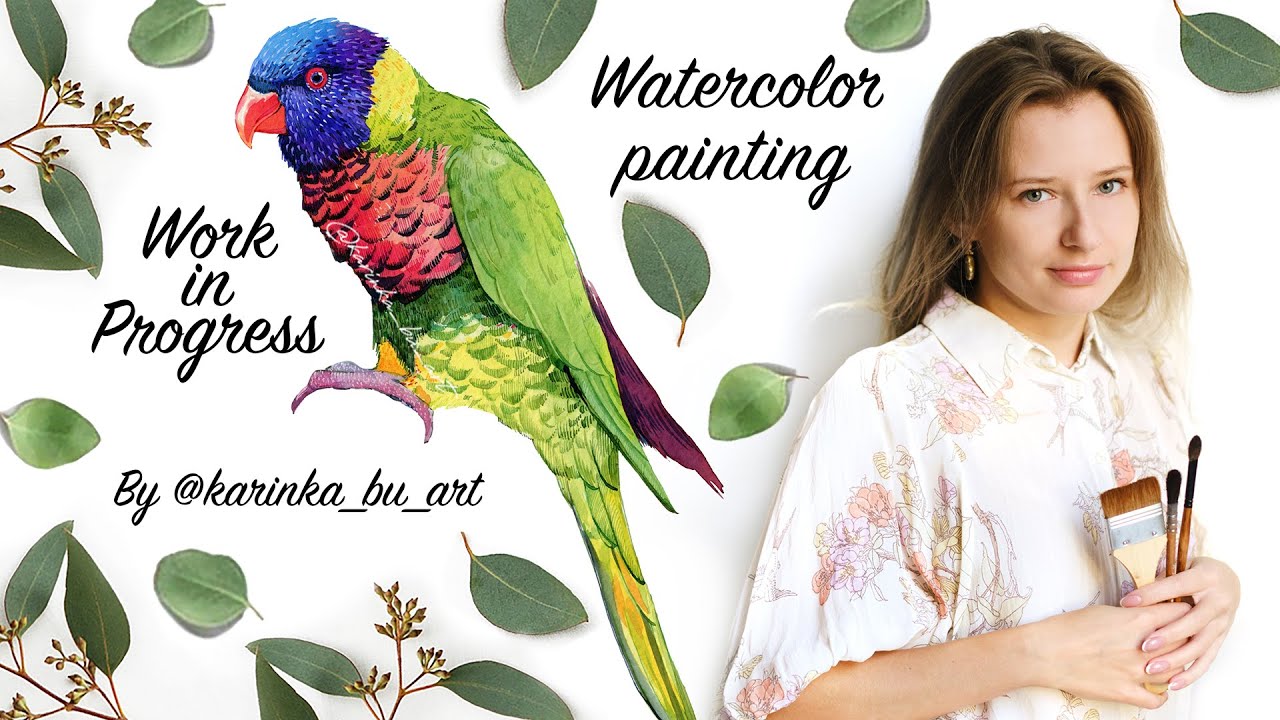The image, set against a plain white background, showcases a detailed watercolor painting of a parrot on the left-hand side and a woman on the right-hand side. The parrot, adorned with a blue head, vibrant green feathers, and a striking red chest, is surrounded by scattered leaves and twigs, adding a touch of nature to the composition. Above the bird, black cursive text reads "watercolor painting," while "work in progress" is inscribed below. 

On the right, the woman, who is of Caucasian descent, has shoulder-length brownish-blonde hair parted in the center and is wearing a white button-up blouse with a floral print. She holds a variety of paintbrushes – one wide and flat, and two thin and long – in front of her chest with her pink nail-polished hands. She has light brown hair, blue eyes, earrings, and pink lips, and gazes directly at the viewer with a slight smile. The artwork is signed "by @Karina_bu_art" beneath the parrot.